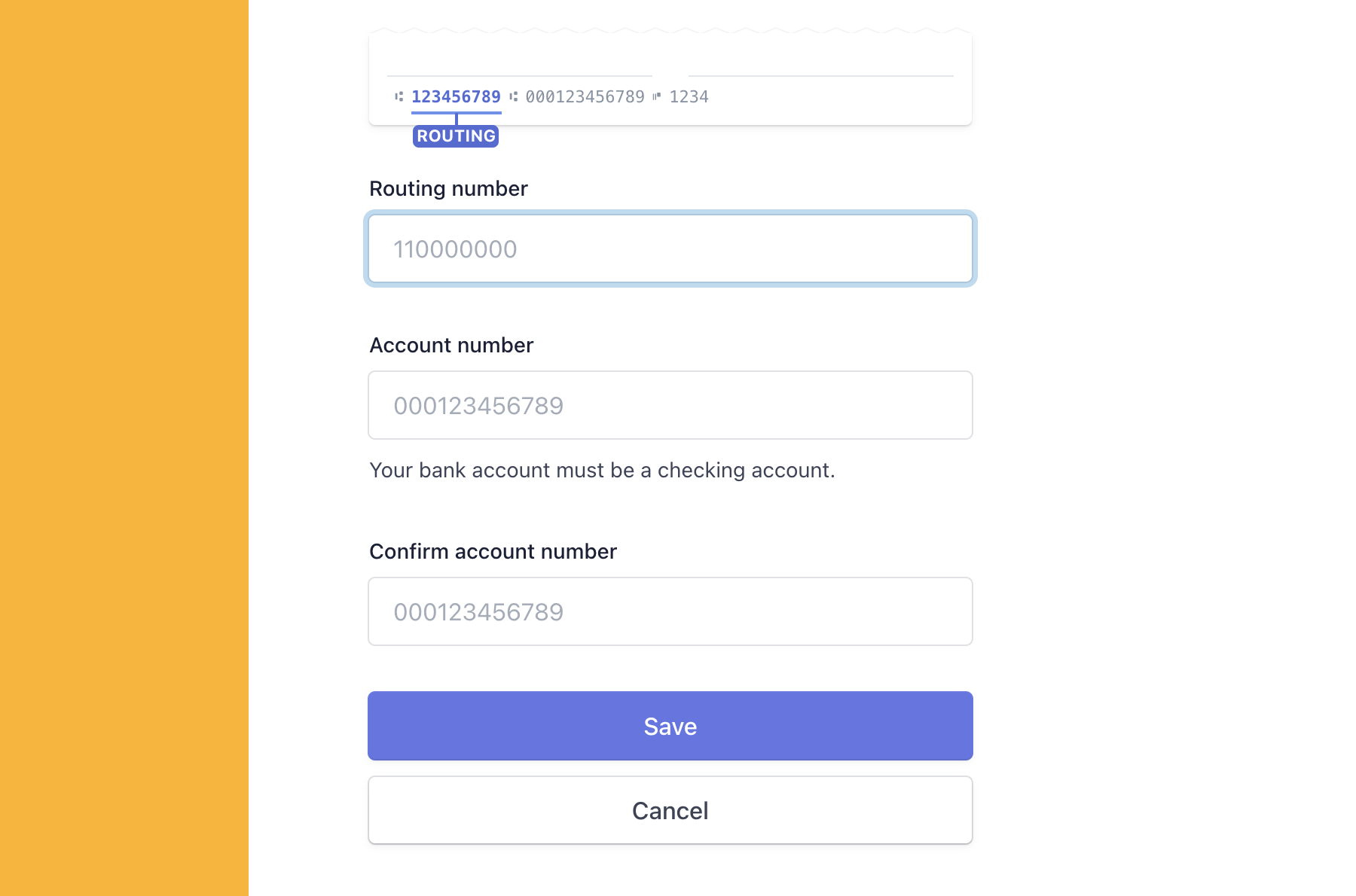This image displays a banking account detail form with a distinct layout featuring a white and yellow design. 

The left portion of the image is colored yellow, occupying around 30% of the space, while the remaining right section, approximately 70%, has a white background. The form is divided into five separate fields:

1. **Routing Number Field**: 
   - Label: "Routing Number"
   - Value: 12345678000123456789
   - The routing number is highlighted with the word "Routing."

2. **Second Field (Routing Number Confirmation)**:
   - Label: "Routing Numbers"
   - Value: 110000000

3. **Account Number Field**:
   - Label: "Account Number"
   - Value: 000123456789
   - Text beneath the box: "Your bank account must be a checking account."

4. **Confirm Account Number Field**:
   - Label: "Confirm Account Number"
   - Value: 000123456789

5. **Action Buttons**:
   - Blue button with white text: "Save" (SAVESAVE)
   - White button with the word: "Cancel"

The form is neatly organized, ensuring clarity in the layout and identification of important banking details.